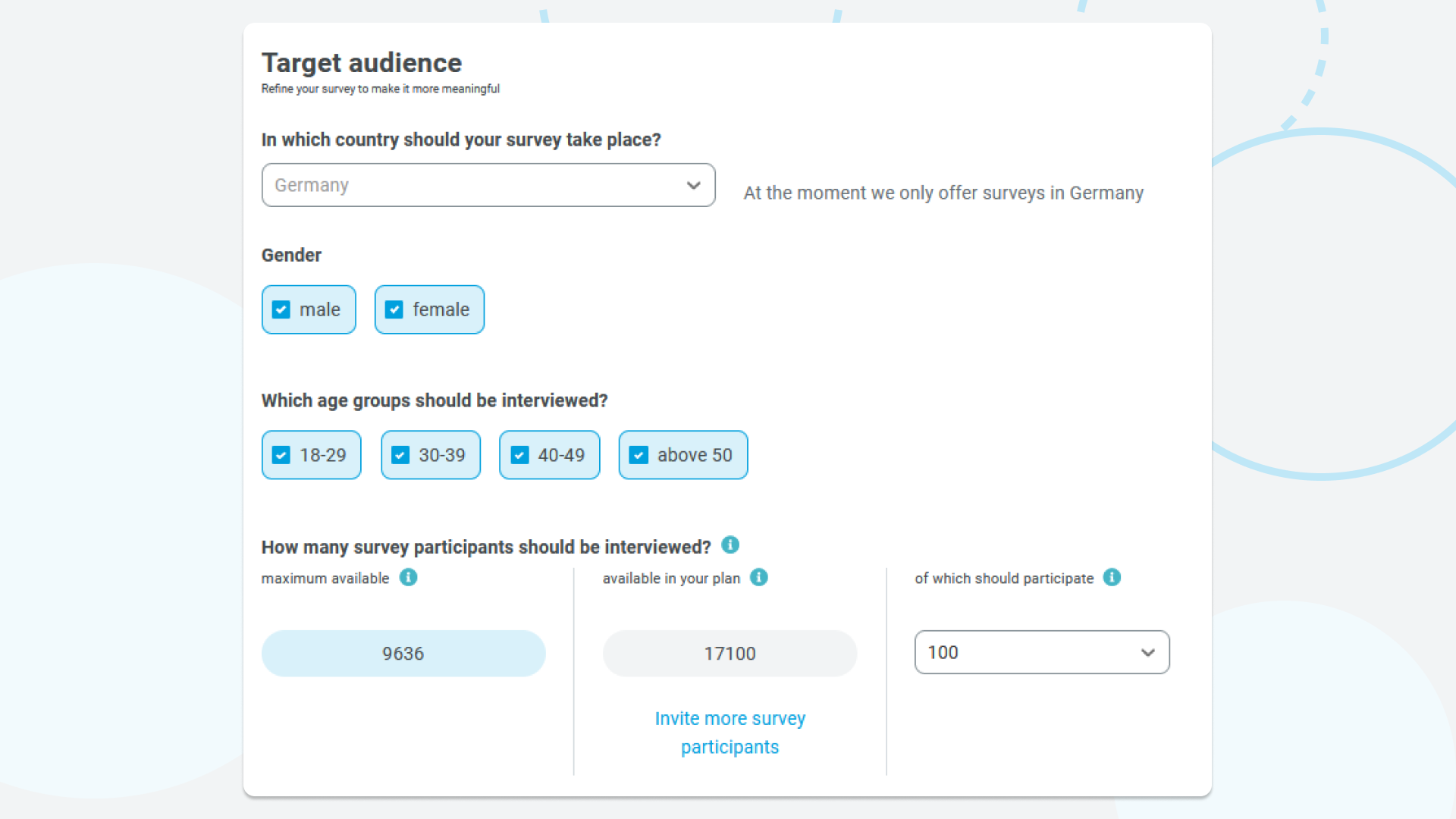The image features a light gray background with various blue circles scattered throughout, adding a touch of visual interest. On the right, a solid blue circle stands out, while above it floats a dotted blue circle. Faded blue circles are situated below and to the left, creating a layered effect.

Centrally positioned is a white rectangular box containing key information. The left side of the box features black text that reads, "Target Audiences." Beneath this heading, in very small font, it says, "Refine your survey to make it more meaningful." Below this, in thicker black font, the question, "In which country should your survey take place?" is prominently displayed. 

A gray outlined box with gray lettering appears next, indicating "Germany" with an arrow pointing to the right. Just outside the box on the right, there is a note in black text that reads, "At the moment, we only offer surveys in Germany."

Further down, the section titled "Gender" presents two blue boxes. The first box, with black font, reads "Male," and features a white checkmark within a bluer box. The second box reads "Female," similarly featuring a white checkmark in a blue box.

The subsequent line asks, "Which age group should be interviewed?" and is followed by four blue boxes each marked with a white checkmark. These boxes represent different age ranges: "18-29," "30-39," "40-49," and "above 50."

Next, the text "How many survey participants should be interviewed?" is indicated, accompanied by a blue circle with a white "i" in the middle. Below this, smaller text reads, "Maximum available," followed by a pale blue circle displaying the number "9636." This is separated by a gray line from the next set of information which reads, "Available in your plan," showing a gray circle with "17,100" inside it. Below this, in blue text, it says "Invite more survey participants," which is also separated by another gray line.

The final section reads, "Of which should participate," next to a blue circle with a white "i." Inside a black-outlined box, the number "100" is listed, accompanied by an arrow in black pointing downwards to the right of it.